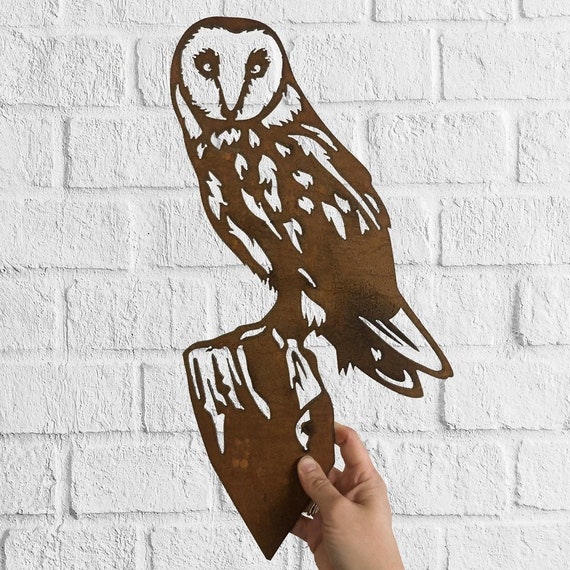The image features a detailed depiction of an owl made from a cut-out metal sheet, possibly crafted using a 2D plasma printer. The metal has a rusty brown appearance, and its intricate design includes white sections where the metal is cut out, revealing the white brick wall behind it, adding an illusion of the owl having a snowy white face. The owl is perched on a similarly styled rock, being held up by a hand emerging from the bottom of the image. The hand, likely that of the artist, is positioned palm facing the left, underlining the handmade nature of this artwork against a uniformly painted white brick background. The transparency and intricate cuts create a compelling visual effect, as if the artwork blends seamlessly with its whitewashed surroundings.